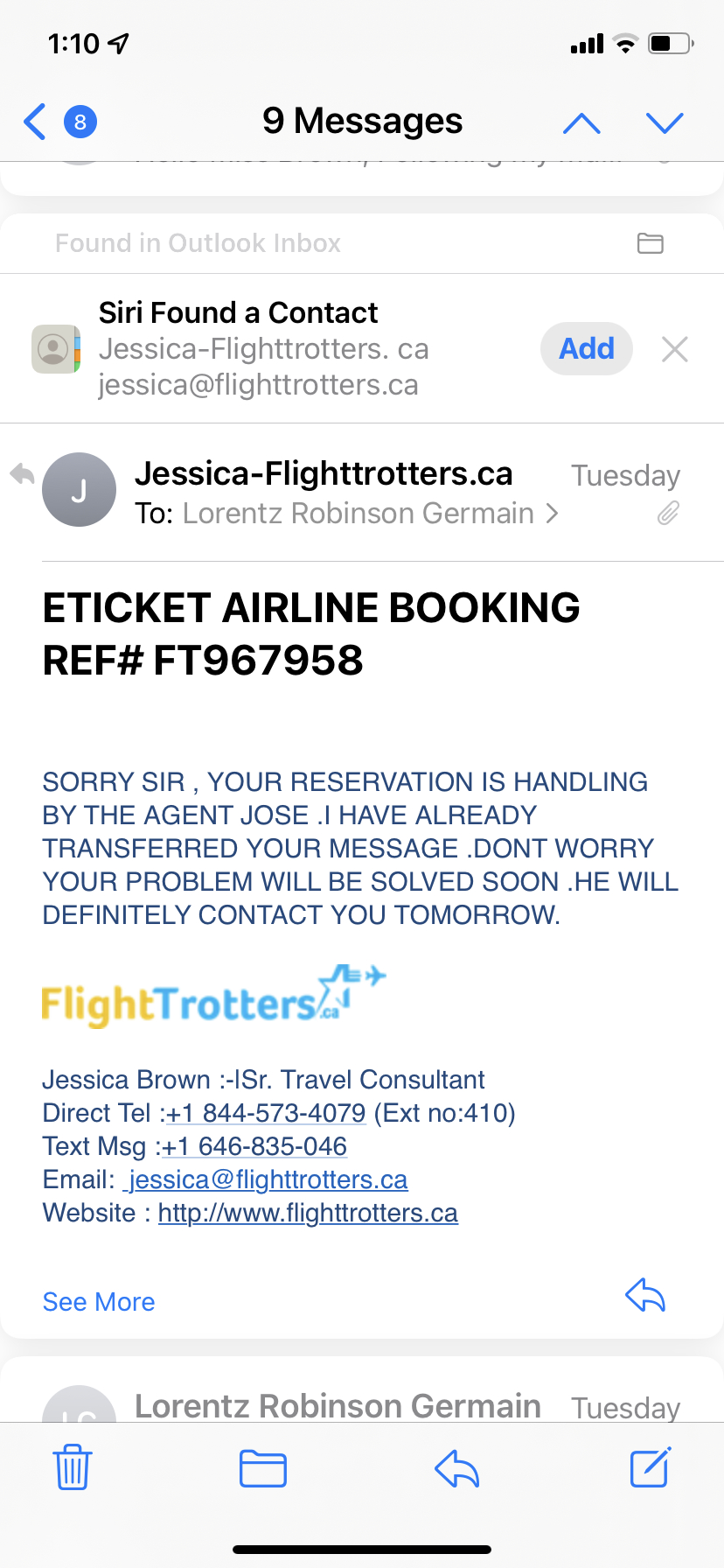This image depicts a smartphone screen displaying various notifications and messages. At the top, the status bar shows 9 messages, a light gray background, and a battery life at approximately 50%. Connectivity icons are visible, and blue arrows indicate data sync status on the right side.

The screen displays the time as 1:10 PM, accompanied by a blue circle with the number 8 inside and an adjacent right-pointing arrow. Among the notifications, there's an alert stating "Found an Outlook inbox" and another informing that Siri has located a contact named "Jessica Fighter Trotters," represented by a generic gray profile picture.

Further down, an additional contact represented by a gray letter 'J' profile picture is shown, identified as "Jessica Flight Trotters." She is engaged in a message conversation with "Lorenzo Robinson, German." The message thread reveals details about an e-ticket airline booking reference number FT 967 958, with text: "Sorry sir, your reservation is being handled by the agent Jose. I have already transferred your message. Don't worry, your problem will be solved soon. He will definitely contact you tomorrow."

The conversation thread includes a "See more" link for additional content. The message display cuts off the name "Lorenzo Robinson, German" and the word "Tuesday."